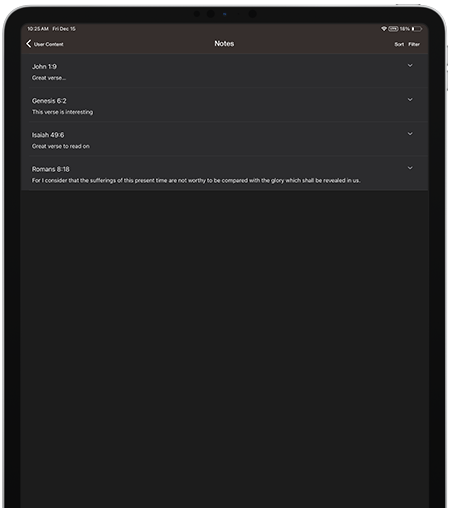This image is a screenshot of a cell phone displaying a notes application. At the top of the screen is a brownish bar. On the left side of this bar, the time is shown as 10:25 AM, alongside the date, Friday, December 15th. On the right side, Wi-Fi and battery icons are visible, with the battery level indicated at 14%. In the center of this top bar, the word "Notes" appears in white font. To the left of "Notes" is a back arrow icon.

Below the top bar, four items are listed vertically in the main content area of the screen:
1. John 1:9
2. Genesis 6:2
3. Word 49:6
4. Romans 8:18